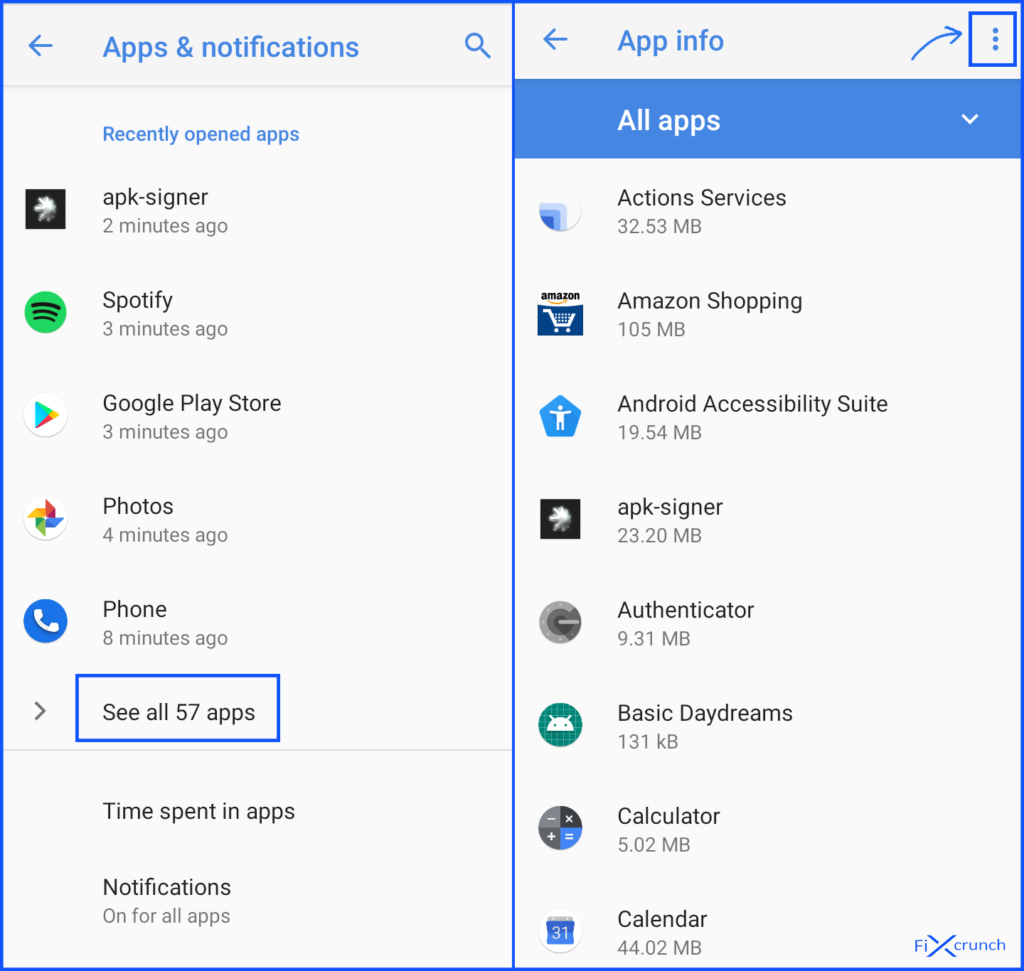This is a detailed image captured from a smartphone's screen, composed of two combined screenshots. 

The top section displays the "Apps & notifications" settings with a continuation into "App info." On the left side, there is a list under "Recently opened apps" which includes icons and names in the following order: DocuSign, Spotify, Google Play Store, Photos, and Phone. The usage time for the app "Phone" is indicated as eight minutes ago.

A blue rectangle, drawn by someone, highlights the text "See all 57 apps." Below this section, the header "Time spent in apps and notifications" is visible with a setting toggle described as "On for all apps."

In the right section, "App info" is displayed at the top with a hand-drawn arrow pointing to the three vertical dots representing a menu. When expanded, this drop-down menu is labeled "All apps." The list of apps within this menu includes names such as Actions Services, Amazon Shopping, Android Accessibility Suite, APKSigner, Authenticator, Basic Daydreams, Calculator, and Calendar. Each app entry is accompanied by its respective icon and specifies the memory usage in megabytes (MB).